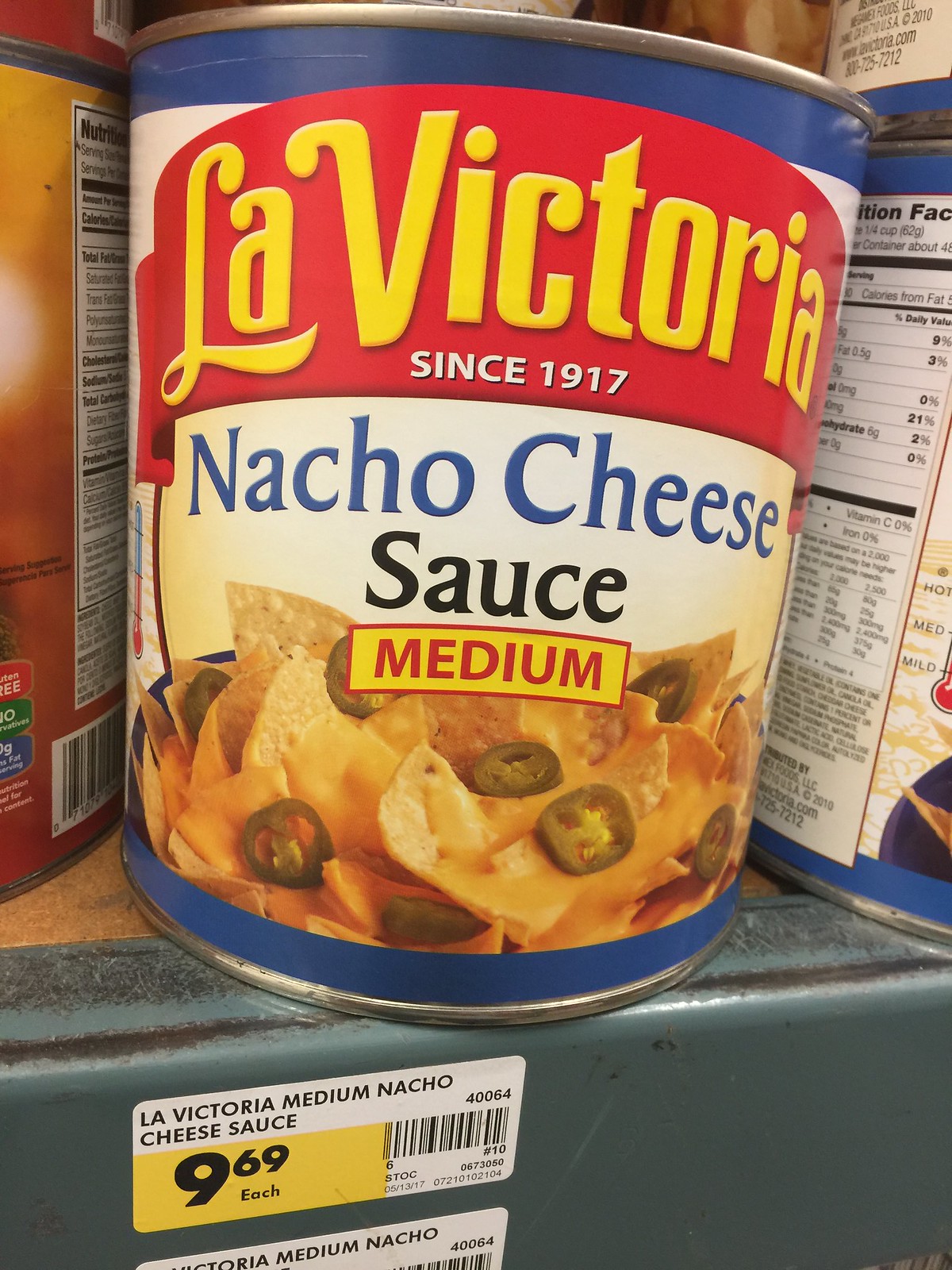This vibrant color photograph features a close-up view of a can of La Victoria Nacho Cheese Sauce. The top of the can showcases the brand name "La Victoria" in bold yellow text set against a striking red banner. Beneath the brand name, it reads "Since 1917" in white font. The main label of the can prominently states "Nacho Cheese Sauce" with the heat level indicated by the word "Medium" in red letters. 

At the bottom of the can's label, there's an enticing photograph displaying crispy tortilla chips generously dipped in nacho cheese sauce, accompanied by slices of green jalapeño peppers, making for a mouthwatering depiction. The can is perched on a store shelf, identified by a label on the side of the shelf that reads "La Victoria Medium Nacho Cheese Sauce" and lists the price as $9.67.